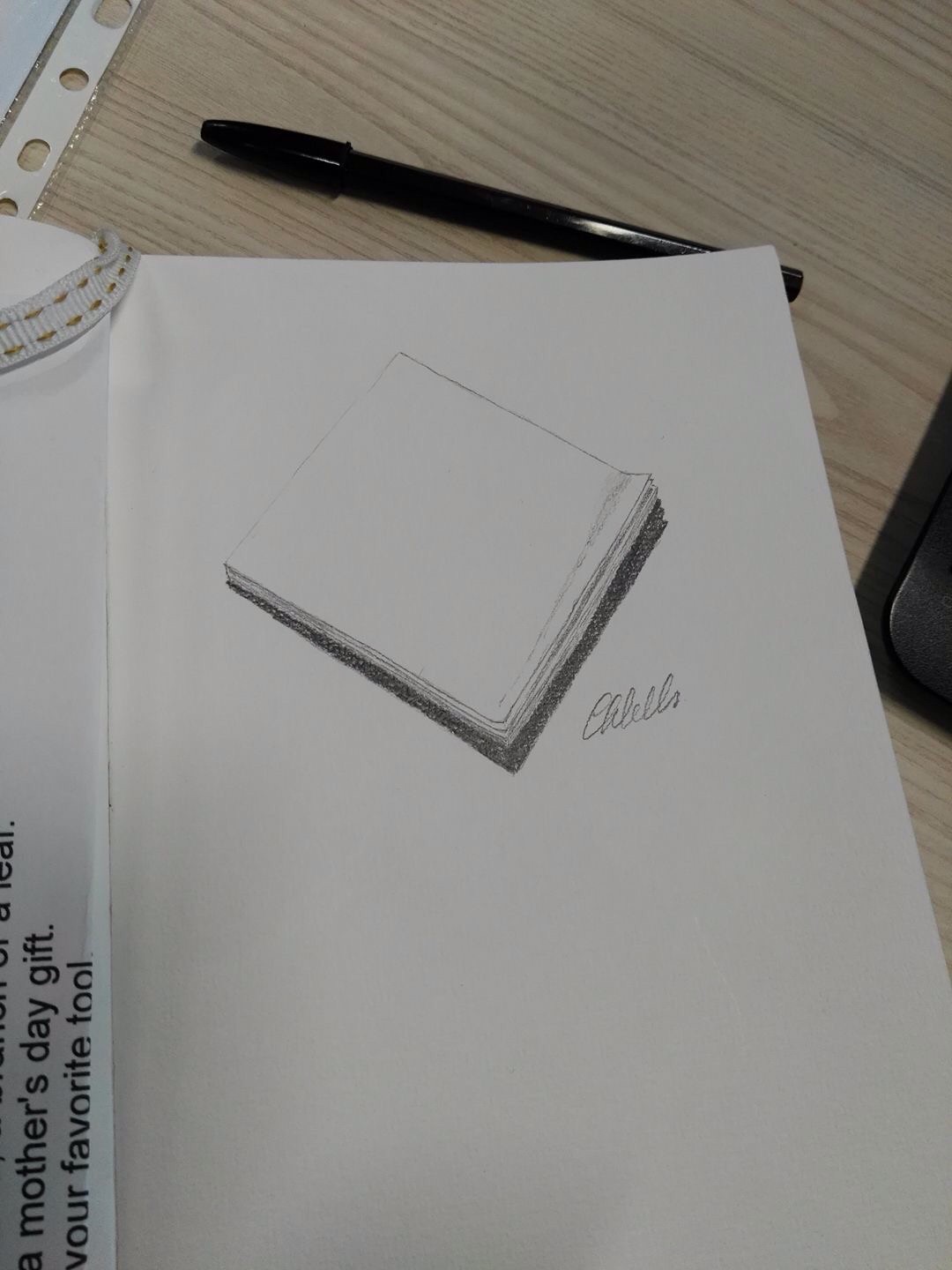A detailed black pencil drawing rests on an open white sketchbook, which is laid out on a blonde woodgrain table or desk. The drawing depicts a stack of paper with meticulously shaded shadows, suggesting slight wrinkles and turned-up bottom edges. These may resemble sticky notes or post-it notes. Underneath the illustration, someone has penciled in their last name, but it remains illegible. Above the sketchbook, a black pen is casually placed on the desk. To the right, the bottom corner of what appears to be an electronic device, possibly a laptop, peaks into view. On the opposite page to the left, there is some black print discussing a Mother’s Day gift.